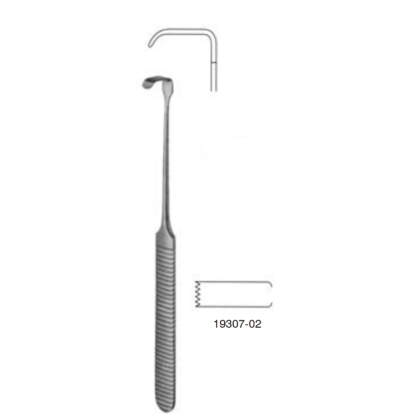This image shows a detailed drawing of an industrial tool, accompanied by a few annotations. The main object in the illustration is a long, dark grey screwdriver positioned vertically on the left side. The screwdriver features distinct horizontal lines along its body and has a black line at its tip. Above the screwdriver, there is a bent L-shaped pipe-like structure, possibly suggesting a thin faucet-like appearance, further extending into a small curve. To the right of the screwdriver, black lines are drawn, resembling electrical resistance symbols, with the code "19307-02" written underneath. The entire illustration is set against a white background, giving it a clean, schematic appearance.